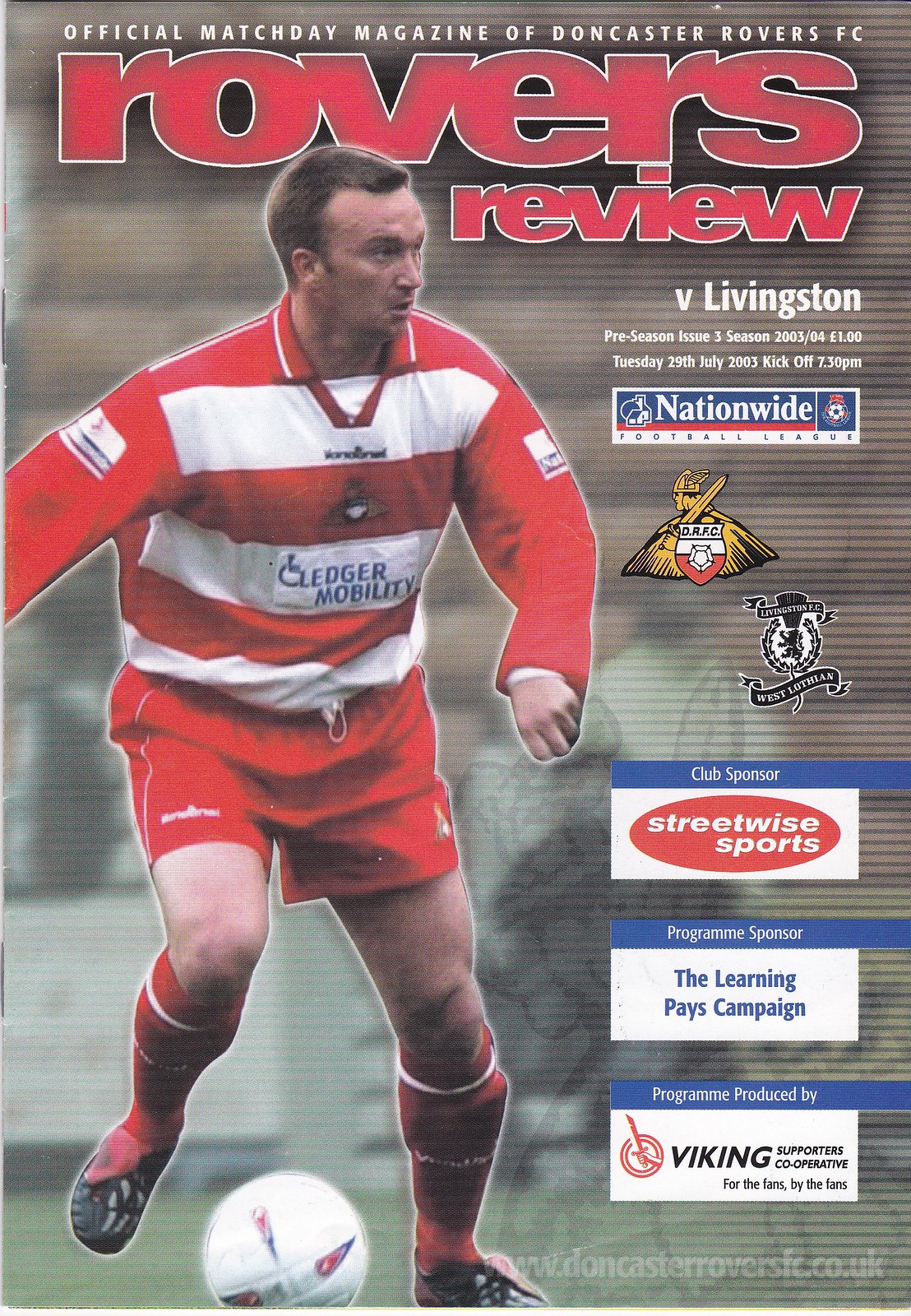The magazine cover, titled "Rover's Review," is the Official Match Day Magazine of Doncaster Rovers FC. The title is prominently displayed in large red text with a thin white border. The edition is the Versus Livingston Preseason Issue, dated Tuesday, July 29th, 2003, for the 2003-04 season, with a kickoff at 7.30 pm, and priced at one euro.

The cover features a dynamic close-up of a Rovers player wearing a red and white striped long-sleeve jersey with the Ledger Mobility logo, red drawstring shorts, red socks with white stripes, knee pads, and red and black soccer shoes. The player is positioned on the left side of the image, mid-action, looking to his right as he kicks a mostly white soccer ball with red and blue accents. The right side of the cover displays sponsorship logos for Nationwide, Streetwise Sports, The Learning Pays Campaign, and Biking, along with other smaller, less legible print details. The background shows the player on an outdoor field, enhancing the motion and intensity of the scene.